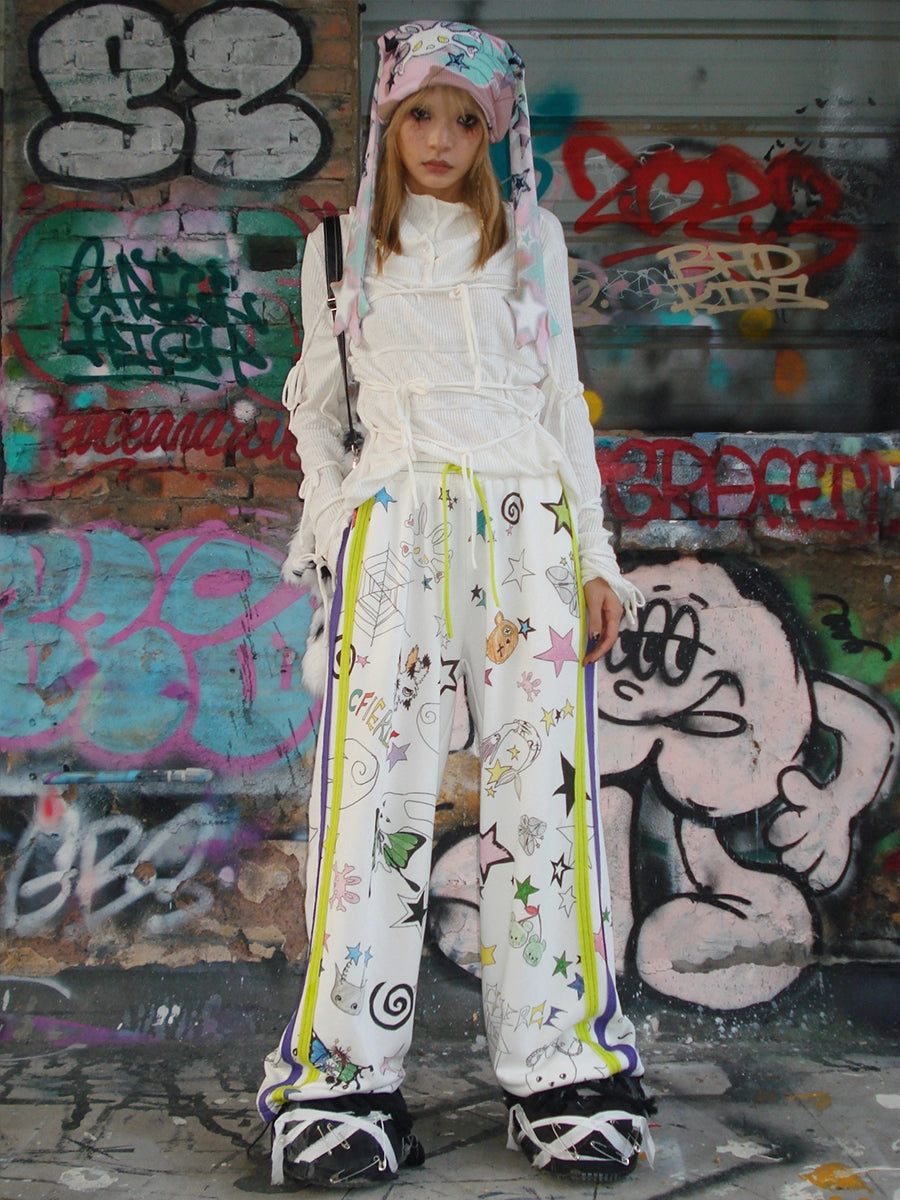The image features a young girl, possibly in an advertisement for hip-hop or street fashion clothing. She stands on a city street in front of a vibrant, graffiti-covered wall displaying an array of colors including white, green, red, pink, and blue, with additional layers of red, tan, and more red on her left side. A noticeable white graphic of a cartoon character occupies the space next to her left leg, extending a third of the way up the wall.

The girl, with her striking blonde hair emphasized by heavy mascara, exudes a distinct fashion-forward vibe. She wears a unique hat, resembling a bunny hat, adorned with pink and blue floppy ears that drape down on either side. Her outfit consists of a long-sleeved white shirt with a textured, patchwork-like design and multiple strings tied across it.

Her white pants, designed in a pajama-like style, are covered in a mishmash of hand-drawn symbols including teddy bears, mermaids, stars, spirals, a cat face, and a spider's web, decorated with colored stripes down the sides—white and black, as well as some yellow. Her right hand is casually tucked into her pocket, and a black bag rests on the same shoulder, partially obscured by her arm.

Completing her eclectic look are oversized, puffy bedroom slippers, intricately crisscrossed with white ribbons over black shiny plastic and seemingly held together with masking tape.